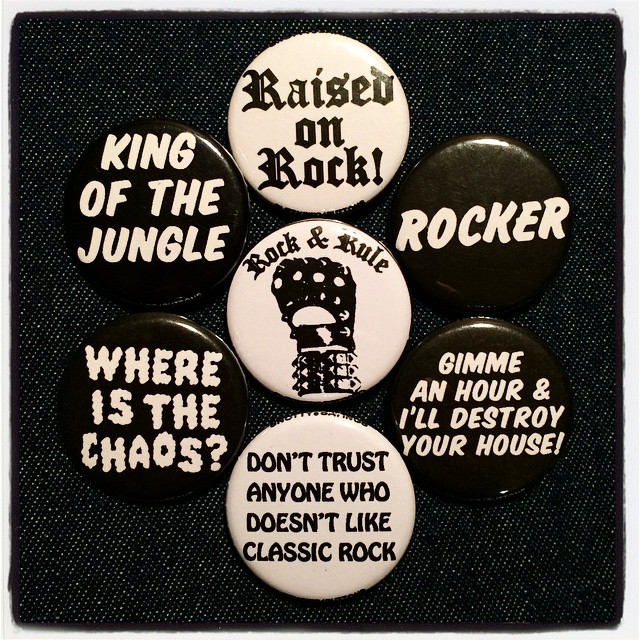The image shows seven circular pins arranged on a background of black denim with small white polka dots and light gray stitching around the edges. At the top left, a black pin in white capitalized letters reads "King of the Jungle," with another black pin below it stating "Where is the Chaos?" in white capital letters. In the middle, two white pins are aligned vertically; the top one says "Raised on Rock" in fancy gothic script, and directly below it, the second pin features a black fist with a cuff and the text "Rock and Rule." Continuing clockwise, a black pin with “Rocker” in bold white print is positioned next, followed by another black pin that declares "Give Me an Hour and I'll Destroy Your House" in white print. Lastly, at the bottom left, a white pin with black letters advises, "Don't Trust Anyone Who Doesn't Like Classic Rock."